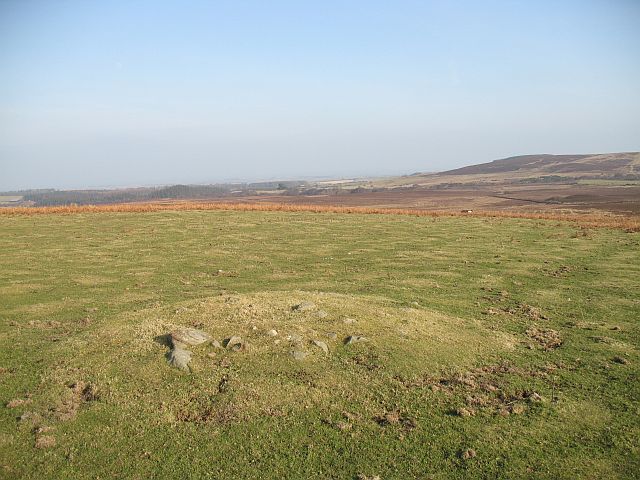This outdoor photograph captures a vast expanse of land, characterized by seemingly endless stretches of green grass interspersed with rocks. At the center of the image, there's a noticeable small mound, presumably the remnants of dug-up earth now covered by overgrown grass and crowned with stones. The rocks appear arranged in a somewhat jagged circular formation, with taller white stones positioned centrally and gray and brown stones surrounding them. The land undulates gently, leading to distant small hills that are green and brown in color. As the landscape extends toward the horizon, a reddish-brown feature, possibly a wall or a different type of hill, comes into view, eventually blending into the beginnings of more prominent, though still modest, hills. The sky above is a light, faded blue, adorned with a scattering of thin, white clouds that add a hazy quality to the distant view. There's a suggestion of a city far off, though no clear structures or inhabitants are visible. The photograph contains no identifying information regarding the location or time of day, leaving an air of mystery about this serene, expansive scene.